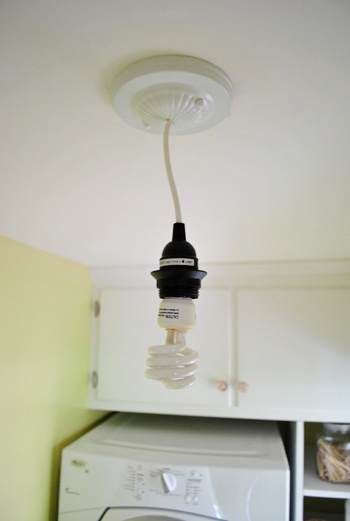The image showcases a detailed view of an energy-saving, cylinder-shaped white LED lightbulb hanging from a black wired cord attached to the ceiling. The top of the cord is visible, leading to an unprotected, downward-hanging lightbulb. The lightbulb features black text and is not turned on. It is set against a background that appears to be a laundry room. On the left, a greenish-yellow wall is visible, while the rest of the room is predominantly white, including the ceiling. In the backdrop, there are two white cabinets with doors, a white washing machine below them, and additional shelving underneath the cabinets. One shelf holds a brown basket. The image focuses primarily on the lightbulb while providing a clear view of the surroundings, indicating a domestic setting with slightly varied image quality.